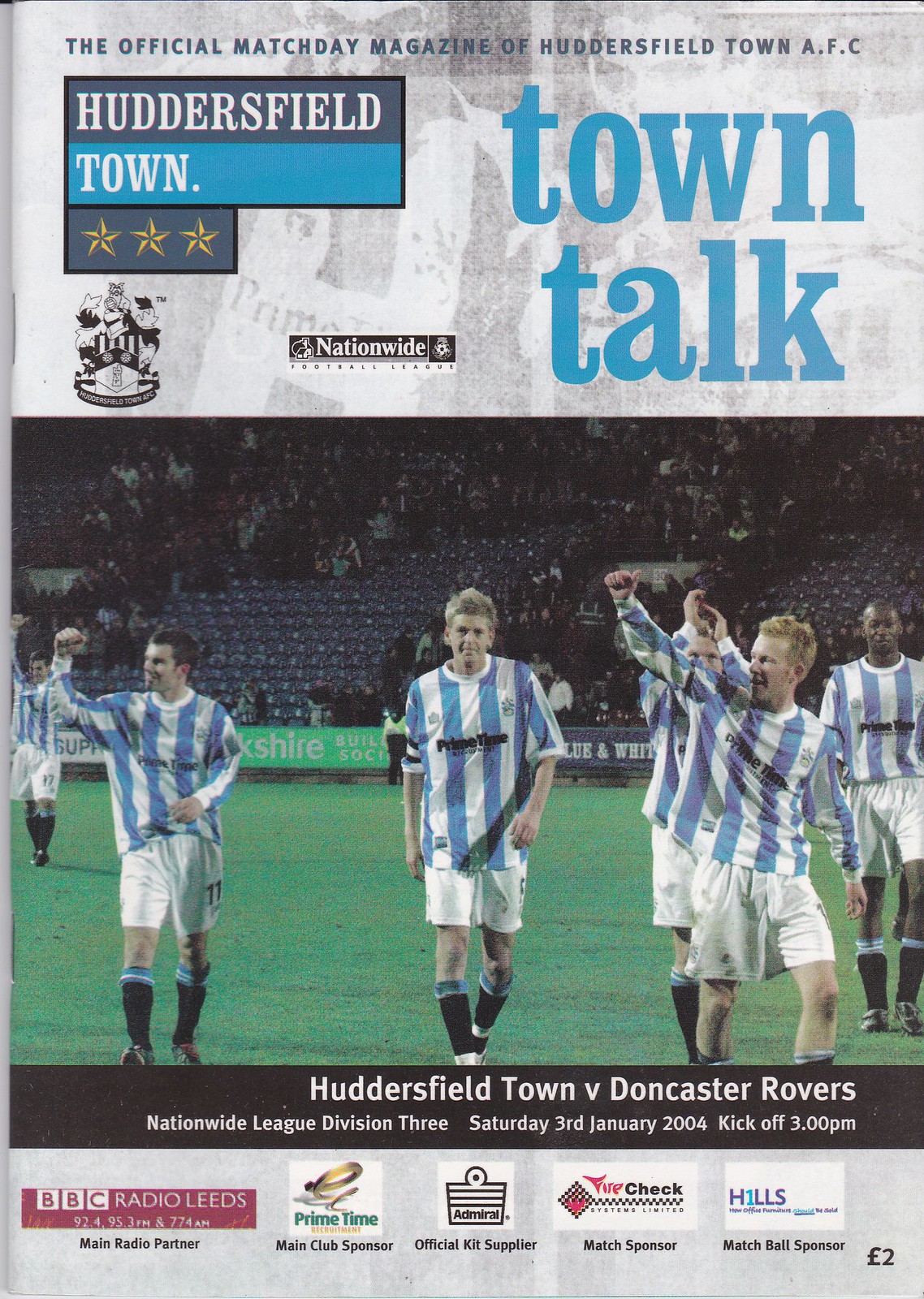This is the cover of the "Town Talk" magazine, the official Match Day publication for Huddersfield Town AFC. The cover features a vertical rectangular layout. 

At the very top, in smaller writing, it reads, "The Official Match Day Magazine of Huddersfield Town AFC." Below that, on the left side, there is a gray box and a blue box with white letters that spell out "Huddersfield Town," accompanied by three stars. On the right side, in large blue letters, is the title of the magazine, "Town Talk."

Dominating the center of the cover is a photograph of the Huddersfield Town team. The players are dressed in blue and white striped jerseys, white shorts, and long black stockings, and they are standing on a green field, many with their arms raised, seemingly in celebration, possibly after winning a match.

Toward the bottom of the cover is a black banner that reads, "Huddersfield Town versus Doncaster Rovers, Nationwide Division 3, Saturday, 3rd of January 2004, kickoff 3pm." Below this, the sponsors are listed, including BBC Radio as the main radio partner, Primetime as the main club sponsor, Admiral as the official kit supplier, and Hills as the Match Bowl Sponsor.

Additionally, the cover features two logos: one placed above the picture in the center, which reads "Nationwide," and another logo, details of which are less clear, positioned below the blue box on the left side.